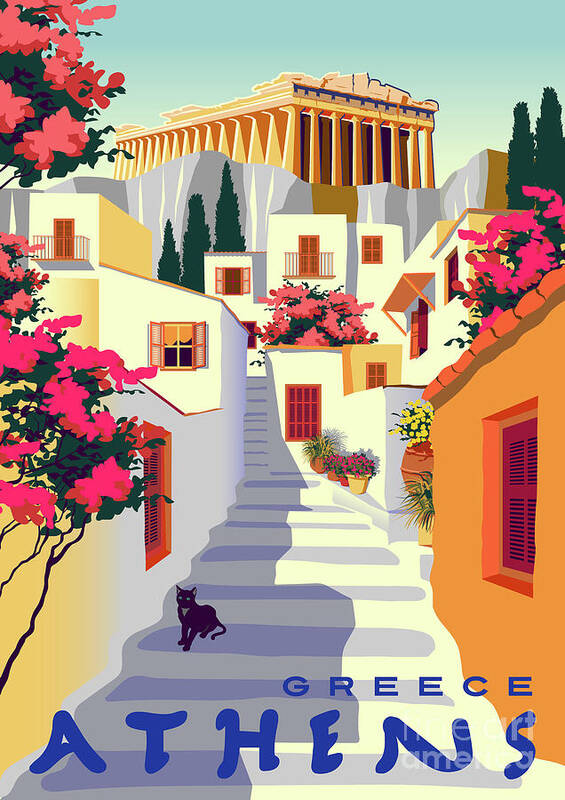The image depicts an illustrated postcard featuring the charming architecture of Athens, Greece. Central to the scene is a stairway leading straight up to beautifully illustrated buildings, adorned with balconies and open windows, with the historical Acropolis visible in the distance. A black cat is perched slightly to the left on one of the steps, adding a touch of life to the setting. The postcard bursts with vibrant colors, including shades of orange, red, maroon, yellow, white, and blue. Red and yellow flowers, fuchsia bushes, and abundant greenery flank the stairs on both sides, continuing along the center. Decorative pottery pots with plants are arranged on the right side of the steps. The houses on either side of the stairway are primarily white or orange with dark red windows, and two trees can be seen towards the top right. A grand, yellow cathedral-like building dominates the background beneath a clear, light blue sky. The text at the bottom of the postcard reads "Greece, Athens" in blue letters.